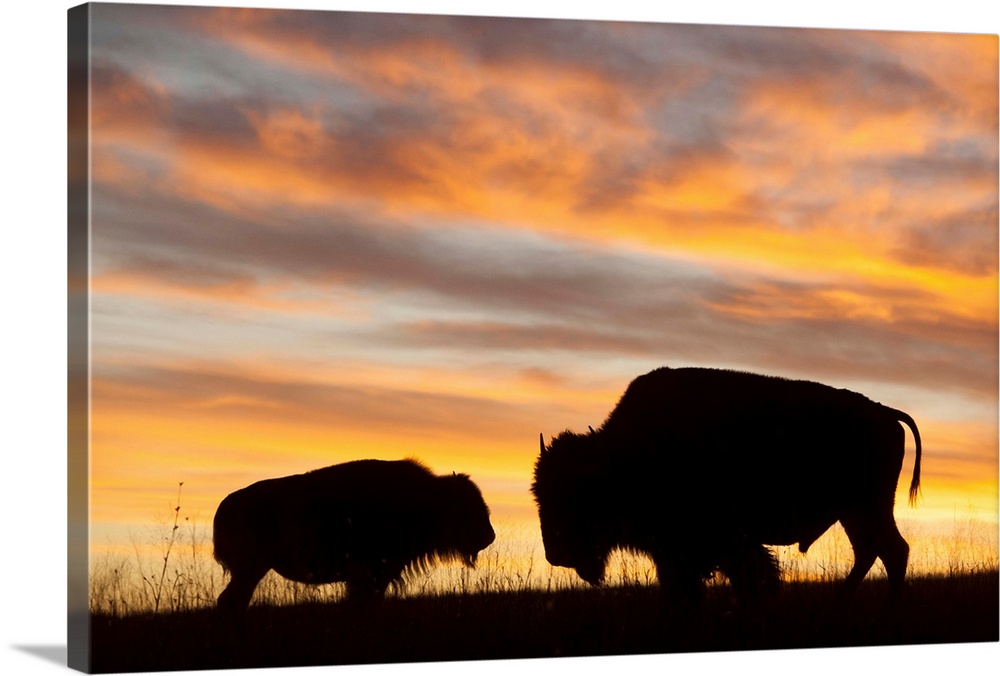The image, presented in a landscape layout with sides shorter than the top and bottom, captures a serene scene at either sunrise or sunset. The bottom 10% of the image appears black due to shadows, but it is likely dark green grass with visible lines of grass and weeds. The backdrop is a mesmerizing blend of hues, including shades of blue, white, orange, pink, yellow, and gray, creating an ethereal sky with swirling clouds and the sun attempting to break through.

In the middle ground, two buffalo – or possibly oxen – face each other, forming a mirrored silhouette. The larger buffalo on the right and the smaller one on the left suggest a parent-offspring relationship. Their detailed forms are lost to the shadows, leaving only their black outlines visible against the radiant sky. The contrast between the silhouetted animals and the vibrant sunset sky enhances the dramatic ambiance of this peaceful landscape scene, amplifying the natural beauty and quiet interaction between the two creatures.